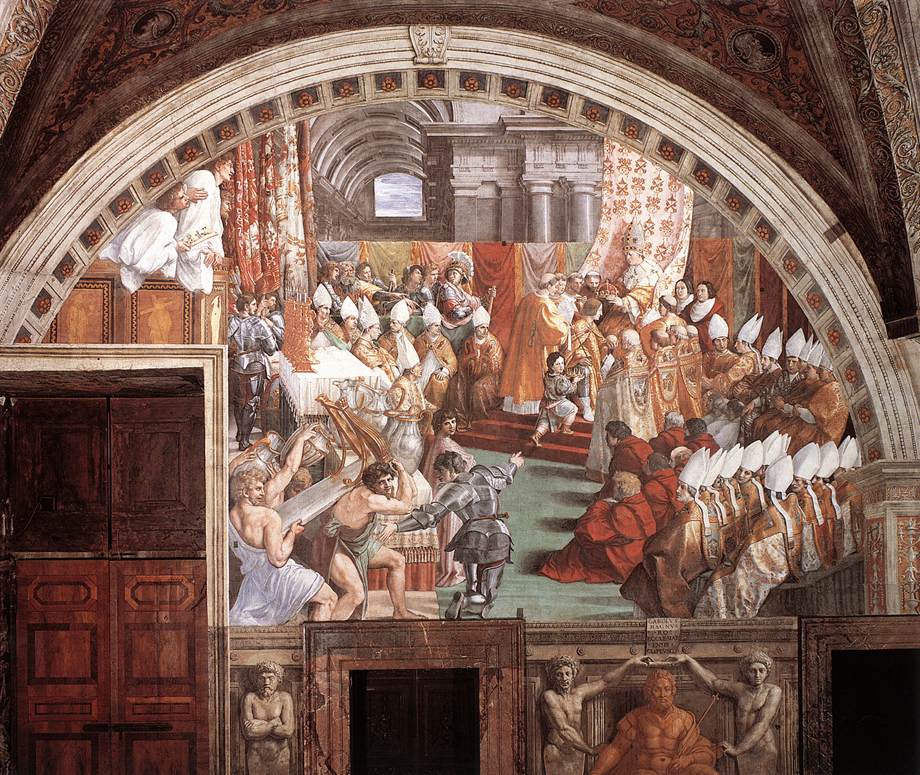This image appears to be a detailed and vibrant painting, most likely set in a Catholic church or religious facility. Dominated by shades of red, brown, tan, black, white, orange, and yellow, the composition features an array of figures and architectural elements that evoke a sense of grandeur and solemnity.

At the center of the painting stands a knight in metal armor, engaged in a dynamic scene that draws the viewer's eye. Flanking him are two men dressed in ancient Roman-style togas, their robes draped over one shoulder. Surrounding this central conflict are numerous clergymen and other figures, including a priest wearing a silver cone-shaped hat adorned with medallions. Some clergy members are depicted in gold and white robes with small caps, while others are seated on the floor in red robes, conspicuously lacking headwear.

Two rows of men wearing gold robes and white cone-shaped hats are also present, seated in a manner that suggests formality and rank. There's an evident youth presence as well, with children interspersed among the adults. The scene is further populated by additional clergy in white cone hats assembled around a table, emphasizing the ceremonial atmosphere.

Architectural details enhance the painting's realism: stone figures adorn the lower part of the image, and a set of ornate wooden double doors suggest an entrance to another sacred space. An overarching arch frames the entire tableau, contributing to the sense of depth and grandeur. The top of the image features exquisite architectural elements that complete this intricate and historically evocative scene.